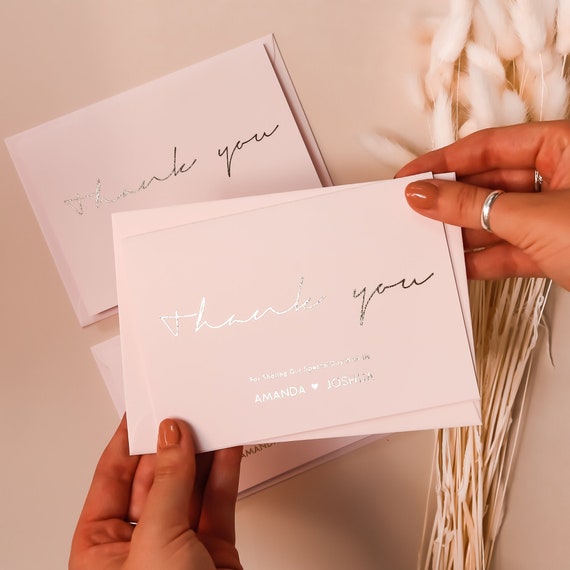The image depicts a pair of hands adorned with three silver rings, delicately holding a thank you card over a cream-colored background with a slight pink hue. The thank you card is elegant white card stock with silver cursive lettering that reads "Thank you" followed by smaller silver print that is difficult to fully discern but suggests a gratitude message, likely for sharing a special day. Below the message, the names "Amanda" and "Joshua" appear with a heart between them. The woman's nails are painted a dark tan and only a portion of her hands are visible. Surrounding the hands is a collection of dried, bleached plants, possibly wheat with cottony tops, arranged in a bundle. Beneath her hands and to the side are at least two identical thank you cards and their envelopes, ready to be sent.